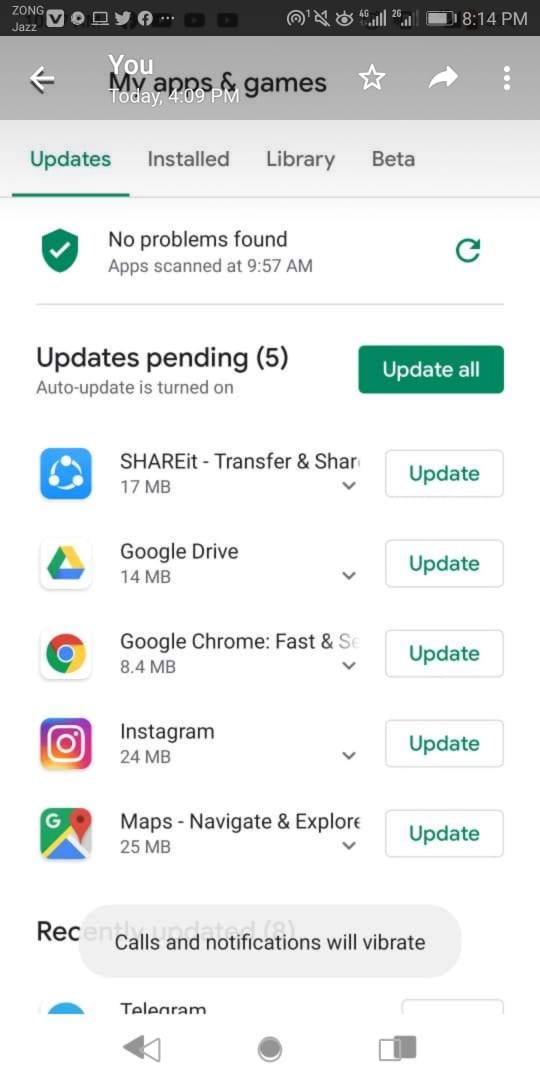This image is a detailed screenshot captured from a cell phone displaying the "My Apps and Games" section of a mobile app store, likely the Google Play Store. 

At the very top of the screen, there is a black status bar which shows various white icons indicating the status and connectivity of the phone. On the left, it reads "Zong Jazz," suggesting a network carrier. To the right, there is a sequence of icons: a square with a 'V' in the center, a gear icon, a computer monitor icon, the Twitter bird, and the Facebook logo, followed by three horizontal white dots. Further right, there is a bullseye icon beside a turned off sound notification button and an eye icon. The signal strength indicators show 4G with full bars, and 2G with three bars. The battery icon to the far right shows it's three-quarters full, and the time displayed is 8:14 p.m.

Below this is a gray navigation banner. In white text, it says "You, Today, 4:09 p.m.". Behind this text, the heading "My Apps and Games" is displayed in black. On the left of this title, there is a white back arrow, while on the far right, there are a white star, a forward arrow, and three vertical dots, indicative of additional settings or options.

The next section, predominantly white, shows various navigation labels with "Updates" highlighted in green and underlined. To its right, other categories such as "Installed," "Library," and "Beta" are listed in black text. Below this, a section with a green shield icon on the left bearing a white check mark indicates "No problems found," with a note that apps were scanned at 9:57 a.m. A green reload button is positioned on the right.

Further down, bold black text indicates "Updates pending (5)," with an "Update All" button in white on a green background to the right. The update list begins with the "ShareIt" app featuring a blue icon, followed by a white "Update" button on the right. Subsequent apps listed with similar formatting include "Google Drive" with its triangular icon, "Google Chrome" with its circular icon and text "Google Chrome: Fast", "Instagram" with its multicolored camera icon, and "Google Maps" with the pin and map icon alongside the text "Maps: Navigate & Explore."

At the bottom of the screen, a wide oval gray button in black text notes that "Calls and notifications will vibrate." Partially visible at the bottom left, the edge of a blue circle hints at the "Telegram" app, noted by text cut off on the right.

Finally, at the very bottom, there are navigation buttons in gray: double back arrows, double circles in the center, and a folder icon labeled with "white sheet" on the right.